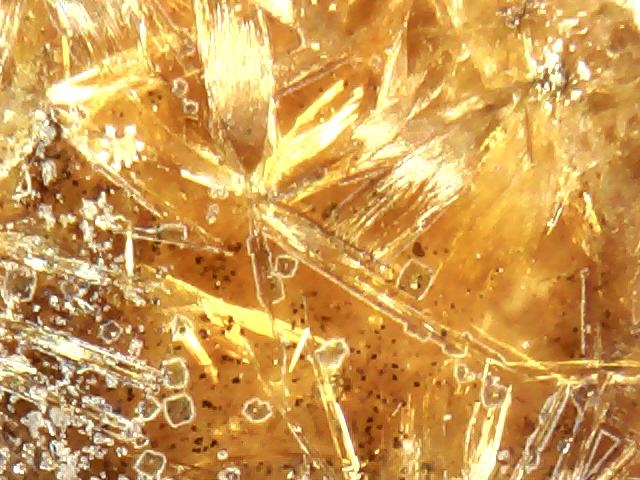The image is rectangular and exhibits a rich tapestry of golds, yellows, and occasional brown hues, creating a bright, shiny scene reminiscent of a crystalline structure or shattered glass reflecting sunlight. This abstract artwork, which might be a photograph, microscope view, or digital rendering, features square shapes and starburst patterns scattered throughout, adding to its intricate detail. The upper left corner reveals brush or paint strokes while the middle to lower left area displays white lines and square shapes. Black specks are sprinkled across the lower central portion. The overall composition evokes the texture of ice cubes in a carbonated drink, with fine cracks and tiny bubbles, further enhanced by the shimmering, warm tones that might hint at a ginger ale or cola. Additionally, some areas resemble the tops of hayseed, adding an organic touch to the geometric and crystalline elements.